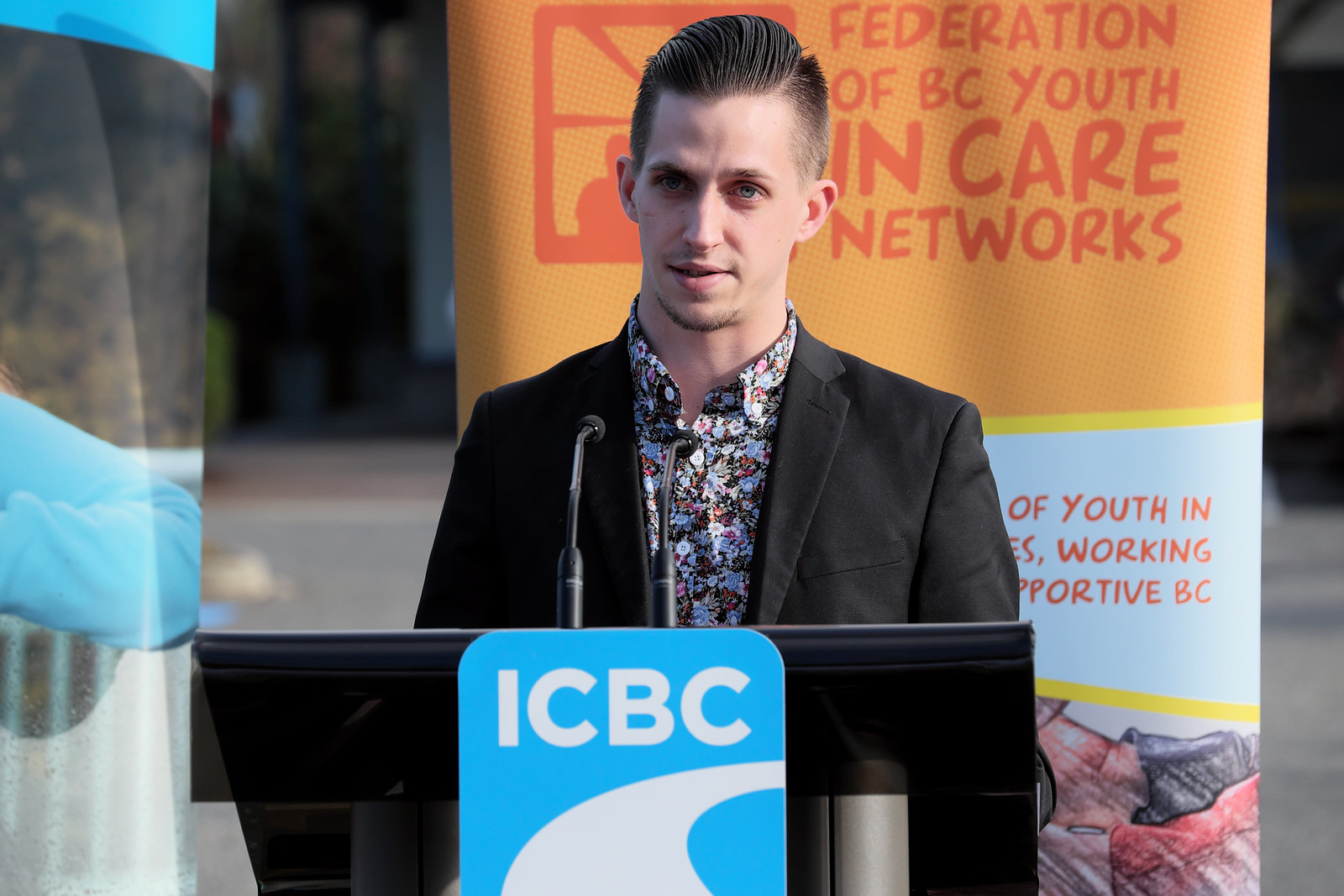In this landscape-oriented photo taken outdoors, a man with brown hair gelled back and parted to the side stands at a black podium bearing a sign with the ICBC logo, displayed in white letters on a light blue square. He has blue eyes and is dressed in a dark sport coat over a colorful buttoned-down floral shirt, featuring small flowers in light blue, purple, and pink. The podium is equipped with two microphones. Behind him is a banner with an orange top portion displaying the text "Federation of BC Youth in Care Networks" in red. Below the orange section, the banner transitions to a blue middle section with partially visible text that reads "Of Youth In" on the first line and "Working" followed by "Port of BC" in red text. The exact location of the photo remains indeterminate.